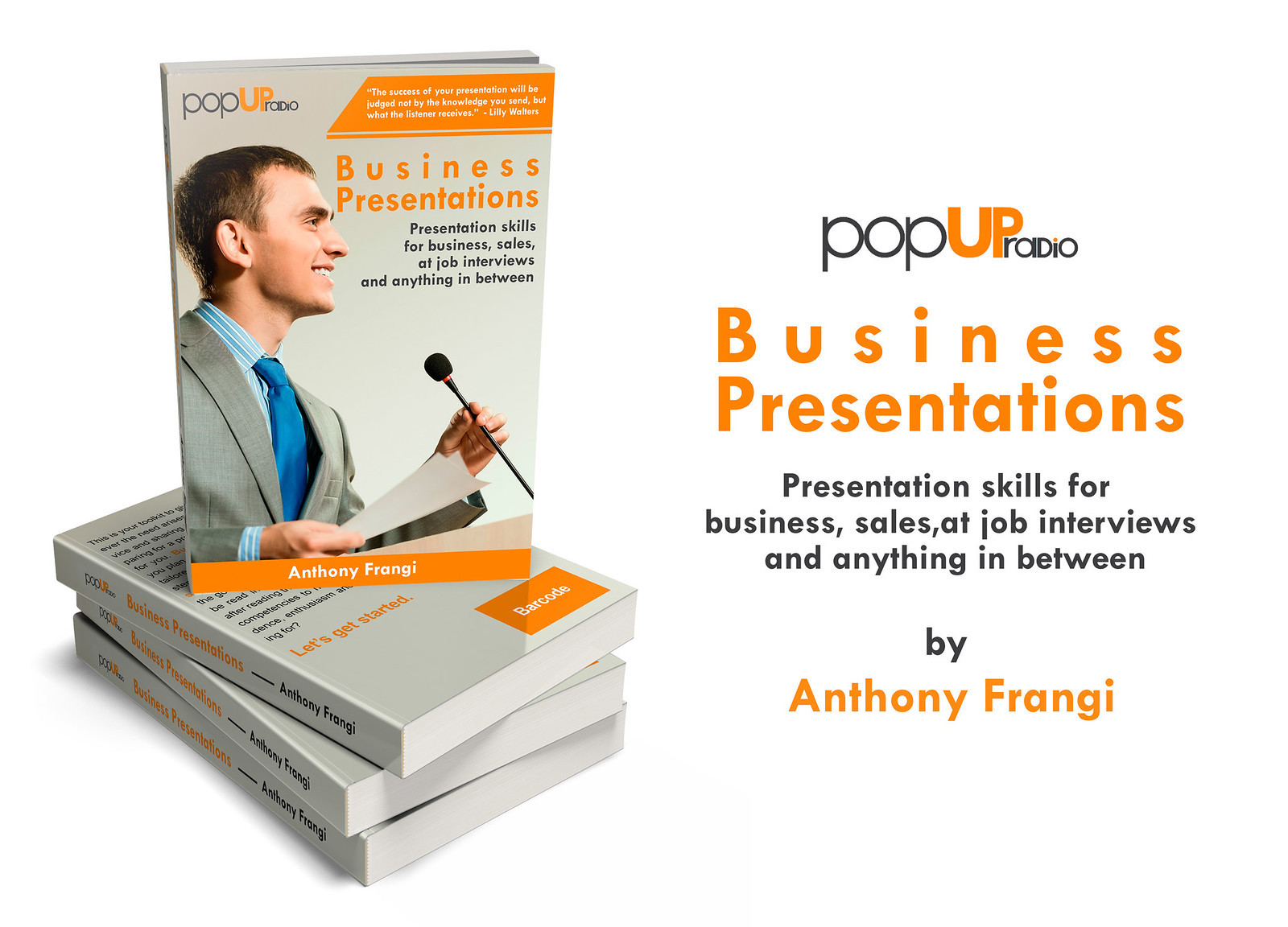The image depicts an advertisement for a book titled "Business Presentations: Presentation Skills for Business Sales, Job Interviews, and Anything in Between" by Anthony Frangie. The setup features four copies of the book, with one propped up on three others that are lying flat on a plain white table. The propped-up book prominently displays its cover, which includes the title in bold orange text and a subtitle explaining its focus on various presentation skills. The cover also features an image of a young man, presumably the author, Anthony Frangie. He is captured standing at a podium, smiling towards an unseen audience while holding a microphone and a piece of paper. Anthony is dressed in a tan sport coat, a white and blue striped long-sleeve shirt, and a blue tie. The background of the book cover incorporates gray, orange, and black elements, creating a professional yet approachable aesthetic.